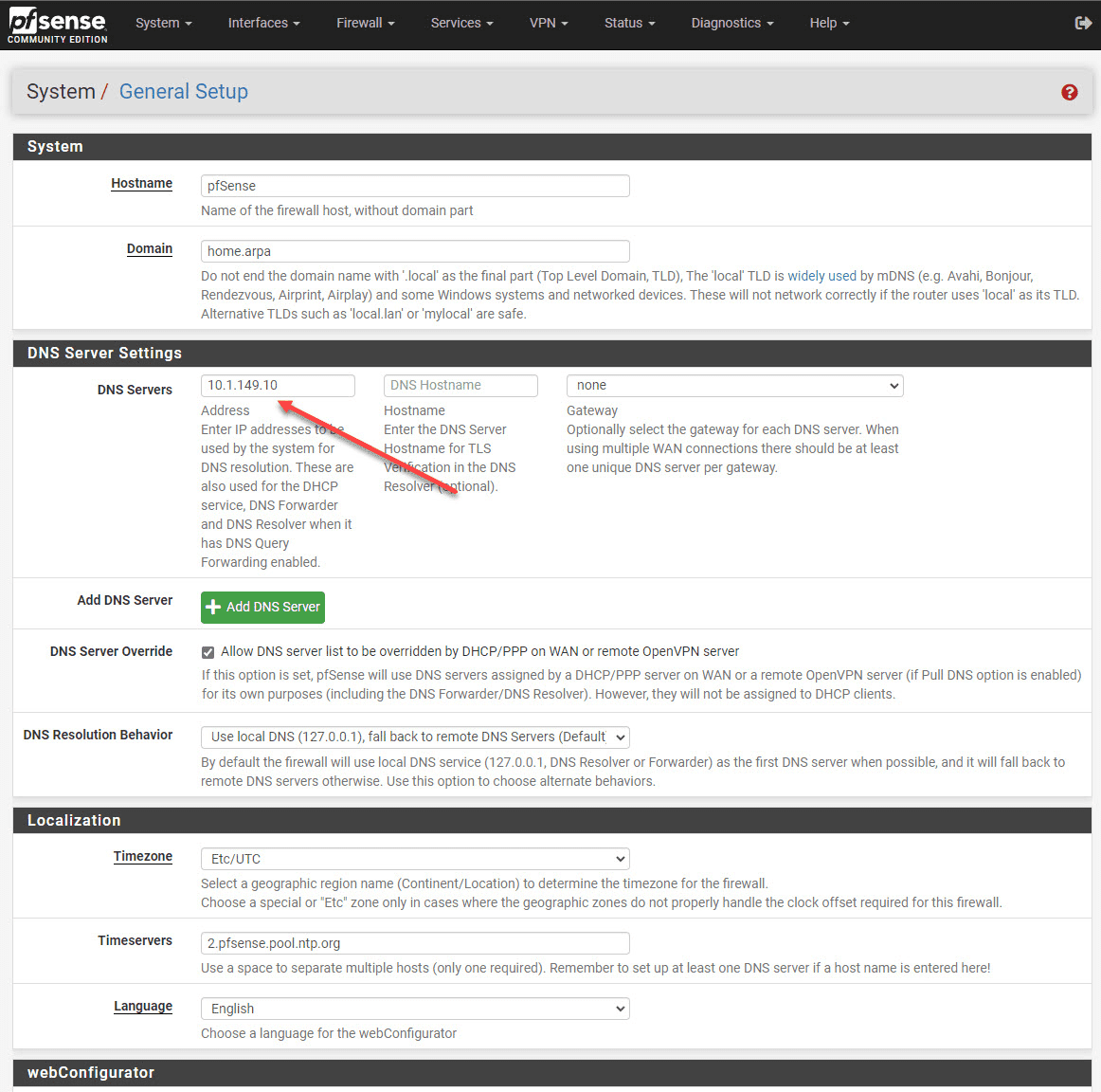The image displays a section of a web interface for pfSense, specifically the general setup page. At the top, there's a black border with white text that reads, "pfSense Community Edition." Below this, there are white tabs labeled: System, Interfaces, Firewall, Services, VPN, Status, Diagnostics, and Help.

Underneath the tabs, there's a long gray rectangle on a white background. On the left side, in black text, it says "System/" and in blue text, "General Setup." On the top right corner of this rectangle, there is a red circle with a white question mark inside it.

A thin gray border demarcates a section where "System" is written in white text. Within this section, the background is white, and various configuration options for pfSense are listed.

The first item under the section is the "Hostname," underlined in black text, with the user-provided value "PDFSense" entered. Below, it specifies "Name of the firewall host, without domain part."

Next, the "Domain" field is underlined in black, showing a partially legible domain that appears to be "hotc.arpa," along with a warning: "Do not enter a domain name with .local as the final part. The local TLD is widely used by mDNS. In some Windows systems and network devices, these will not network correctly if the router uses local as this TLD. Alternative TLDs such as local.dian or my.local are safe."

Further down, there is a section labeled "DNS Server" with an instruction to "Add DNS Server." There is a green rectangle featuring a white plus sign and the text "Add DNS Server," indicating an option to add additional DNS servers.

Overall, the interface is detailed and includes specific instructions and warnings for proper configuration.